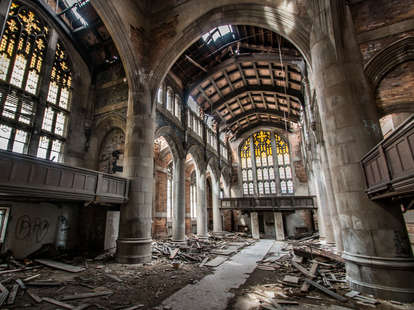This image captures the interior of a massive, centuries-old church now in a state of disrepair. The expansive space is marked by soaring high ceilings and impressive, though muted, stained glass windows that still retain hints of gold and cross motifs amidst predominantly slate gray and concrete hues. The architectural grandeur is further emphasized by enormous, cylindrical columns that rise up, though the overall atmosphere remains dark and somber due to limited sunlight filtering through small holes in the ceiling and the scattered debris on the dirt-covered floor.

Despite the neglect, the high arches and detailed craftsmanship hint at the church's once-magnificent past. Wooden boards and rubble lie strewn across the ground, contributing to the church's desolate and abandoned appearance. The light brown supporting structures show different shades of age and decay, with star-like designs adding subtle elegance amidst the ruins. The photograph, seemingly taken with a professional camera, showcases the forlorn beauty and historical significance of this sanctuary, void of any human presence.